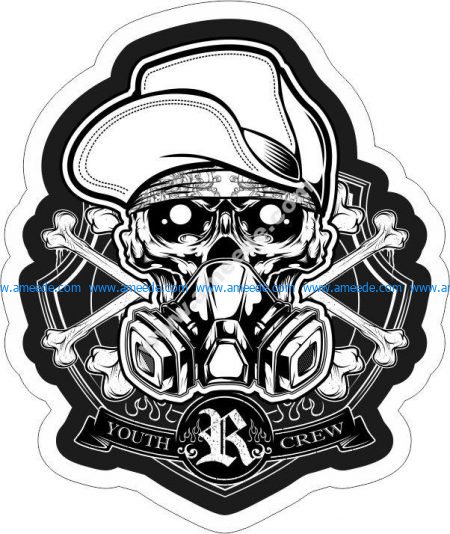The image depicts a uniquely shaped sticker with a white border and a black background, resembling a shield with various dips and curves along the edges. At the center of the sticker is a skull with white dots for pupils, adorned with a sideways ball cap and a bandana visible just beneath the front of the hat. The skull is also wearing a gas mask. Behind the skull, there is a thin pair of crossed bones. Below the skull, a fancy capital letter "R" sits prominently in the center of a ribbon-like banner. The left side of the banner reads "Youth" and the right side reads "Crew," forming the phrase "Youth Crew" around the ornate letter "R."